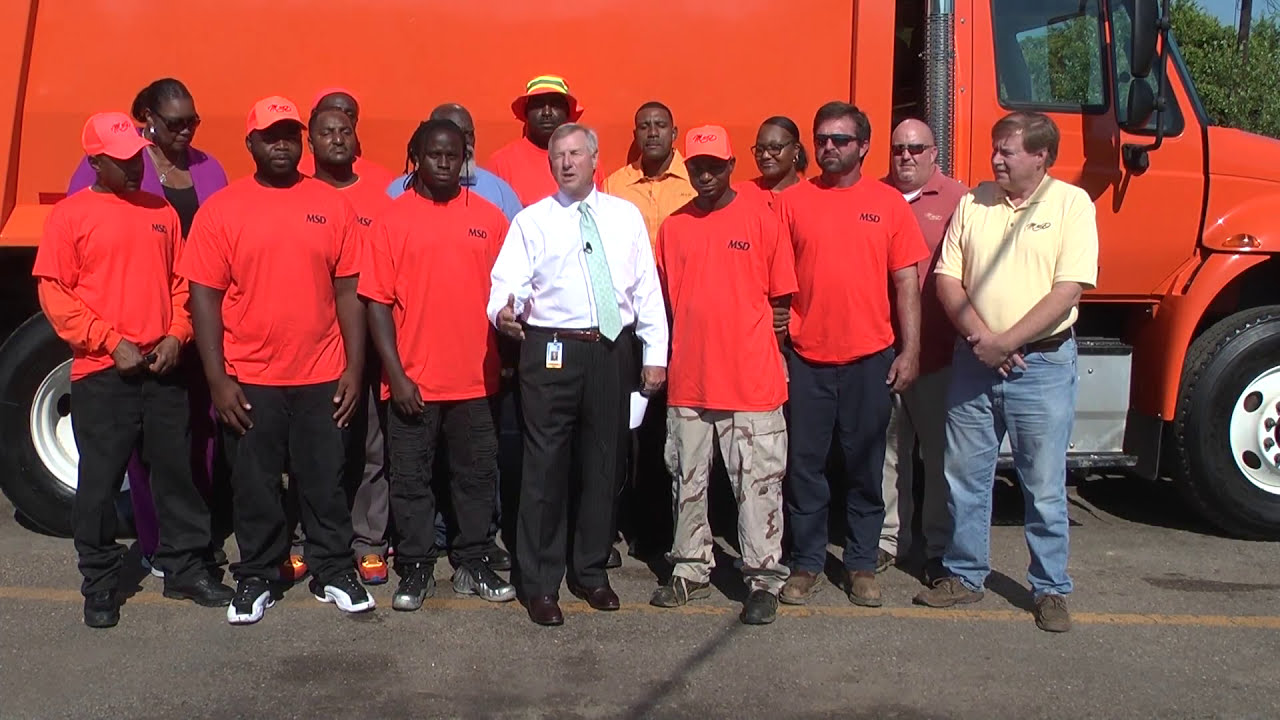The photograph captures a diverse group of people standing in front of a large orange commercial truck, its right side visible facing the camera. The group is positioned on a yellow line painted on the asphalt road. Most individuals are African-American, with a few Caucasian men among them. Prominent in the center is a man with gray hair, clad in a white dress shirt, light blue tie, black pants, and brown shoes. He has a name tag on his belt and a microphone clipped to his tie, suggesting he might be giving a speech or instructions. Surrounding him are people dressed in red shirts with the initials "MSD" printed on the top left corner in black, and some in other brightly colored attire. Of note is a person on the far left with an orange shirt and pink hat, and another on the far right in a yellow shirt and blue jeans. The truck behind them, a bright orange with black tires and white hubcaps, frames the group, contributing to the vibrant color palette of the image. The scene is further characterized by a tall African-American man in the back row wearing a distinctive hat with yellow and gray stripes, and nearby, a green tree is partially visible through the truck's window.